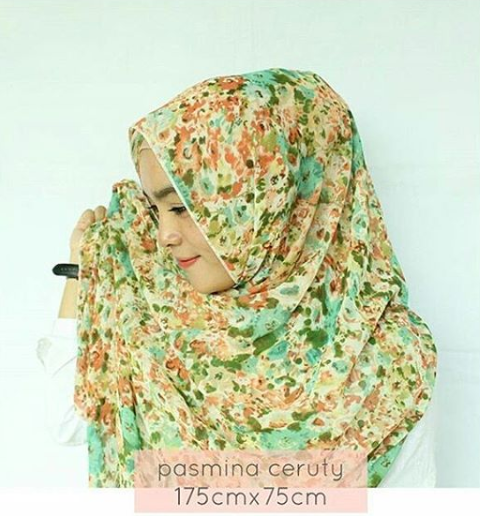The photograph showcases a young woman wearing a colorful, floral headscarf, standing against a light, neutral background, possibly light green or blue. The scarf, adorned with a blend of vibrant colors including various shades of blue, green, turquoise, orange, red, and yellow, is elegantly draped around her head and shoulders. She is positioned at the center of the image, looking to her right with a radiant smile, her makeup done beautifully. Her right hand delicately holds up one end of the headscarf, which highlights the product effectively. She wears a white shirt beneath the scarf and a black wristwatch on her right wrist. At the bottom center of the image, text reads "Pashmina Seruti 175cm x 75cm," suggesting that the photograph is a promotional shot for the headscarf.